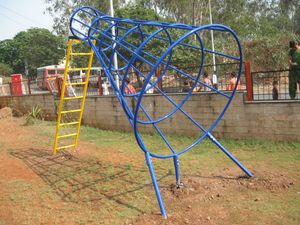In this horizontal rectangular image of a playground, the foreground is dominated by a unique jungle gym structure. This structure appears to be a metallic blue cone with a narrow yellow ladder extending from its top down to the ground. The cone widens as it extends outward from the ladder, allowing children to climb up the ladder and navigate through the metal bars, or to start from the broader end and make their way up to the ladder. Surrounding the base of this structure is a ground covered with patchy grass and reddish dirt.

Behind the jungle gym is a brown brick wall topped with black metal fencing, sectioning off this piece of playground equipment from the rest of the park. On the other side of the wall, several people wearing various colored shirts are walking by. This suggests the presence of a nearby pathway or road. Also visible in the background are trees with green leaves, hinting that the season is either spring or summer. Some orange-colored porta-potties and a red vending machine are positioned near the group of people, adding to the bustling, communal feel of the scene.

Above the image, there's a faint power line crossing over from the upper left corner, and in the distance behind the wall, a bus is visible. This detail, combined with the presence of bystanders and porta-potties, suggests that the location could either be a school playground or a popular tourist destination.